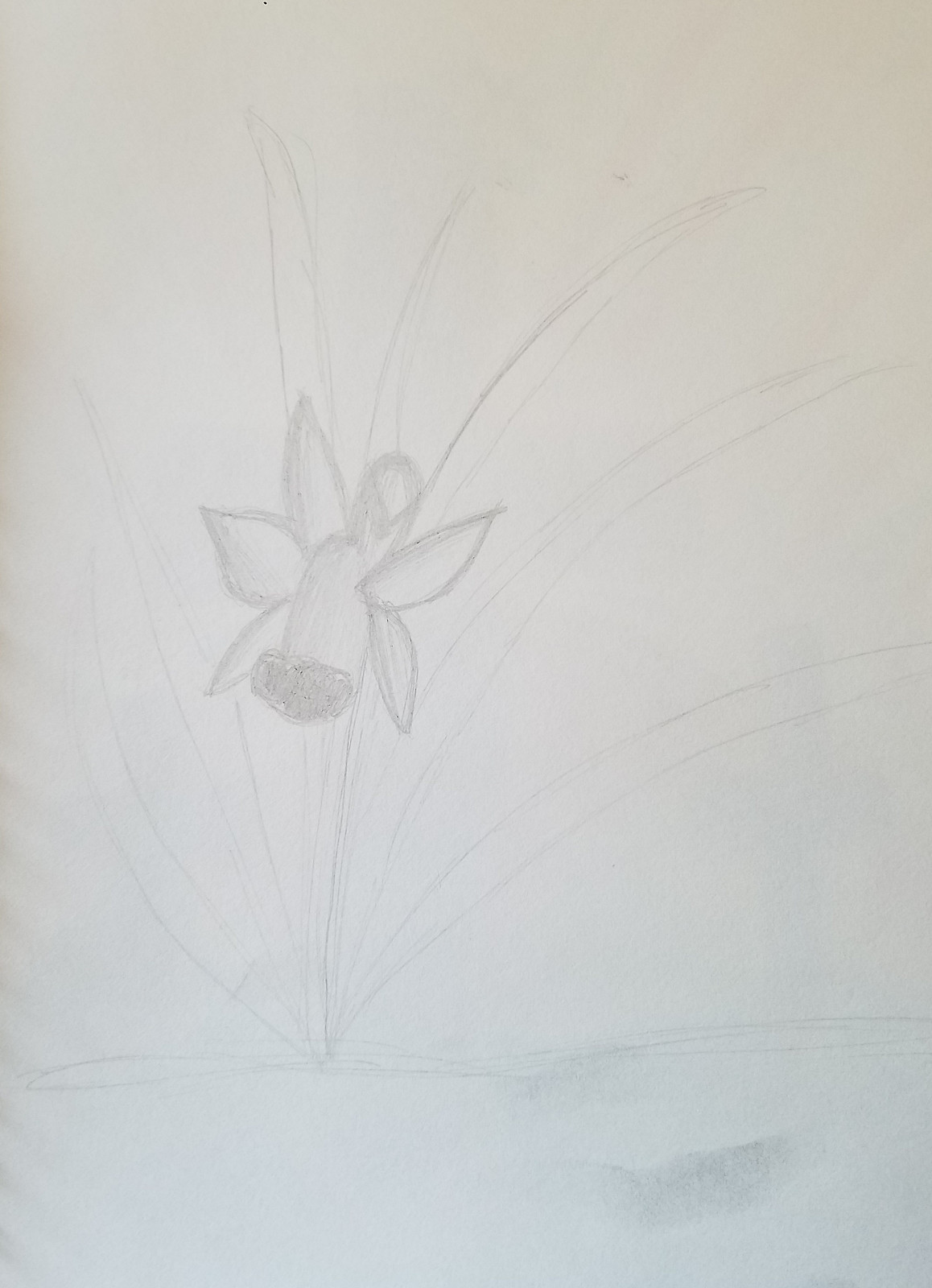The zoomed-in image showcases a detailed pencil sketch on a white piece of drawing paper. The sketch depicts a ground area towards the bottom of the page, illustrated with lines and squiggly marks that resemble dirt or grass. Emerging slightly to the left of the center is a flower with a long stem and large, pointed leaves spreading out from its base. The flower features a tube-like structure, possibly a daffodil, with a shaded, bell-shaped center and five or six petals, some of which could be overlapping or partially hidden. There's noticeable smudging on the bottom right-hand side and faint, pale marks suggesting additional leaves or background details.